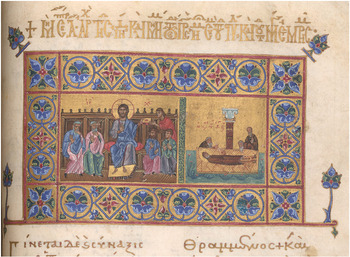The image appears to be an old, intricately designed biblical illustration, rendered on beige-colored parchment paper with a prominent brown hue. The central focus is a rectangular scene featuring Jesus, identifiable by the halo encircling his head, garbed in a grey or blue robe with another blue attire overlay. He is seated with five individuals, two on his left clad in pink, blue, and green, and three on his right wearing a mix of blue, green, pink, grey, and one in red who appears to be passing an object.

On the right side of the image, another prominent scene depicts a person lying on what seems to be a table, with two others beside him. The borders of the illustration are lavishly decorated with geometric shapes, such as rectangles, circles, and kites, and interspersed with floral motifs, predominantly blue in color. The corners of the image also feature blue flowers, both at the top and bottom, lending a cohesive decorative theme.

The top and bottom of the illustration are adorned with gold inscriptions, likely in an ancient or religious script, possibly Latin. The whole piece, reminiscent of a monk's illuminated manuscript, is a testament to detailed ancient artistry with its blend of vivid colors and intricate designs.